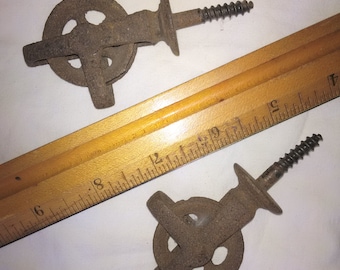The image captures a detailed scene of a worn, antique setting. A diagonal wooden ruler, yellow in color, spans from the lower left to the upper right of the frame, displaying the calibrations from 4 to 9 inches with the numbers upside down. Positioned diagonally opposite to each other on either side of the ruler are two identical, intricately designed metal bolts, appearing dark grey to almost black due to rust and age. Each bolt has a screw end and a pulley-like wheel at the top, signifying a unique, possibly ancient design. The backdrop of the image is a plain, white surface, possibly adorned with a cotton cloth aiding in the display. The lighting is influenced by the camera's flash, highlighting the textures and details of the rusty bolts and the calibrations on the ruler. This meticulously measured arrangement suggests an intent to showcase the dimensions and detail of these artifacts.